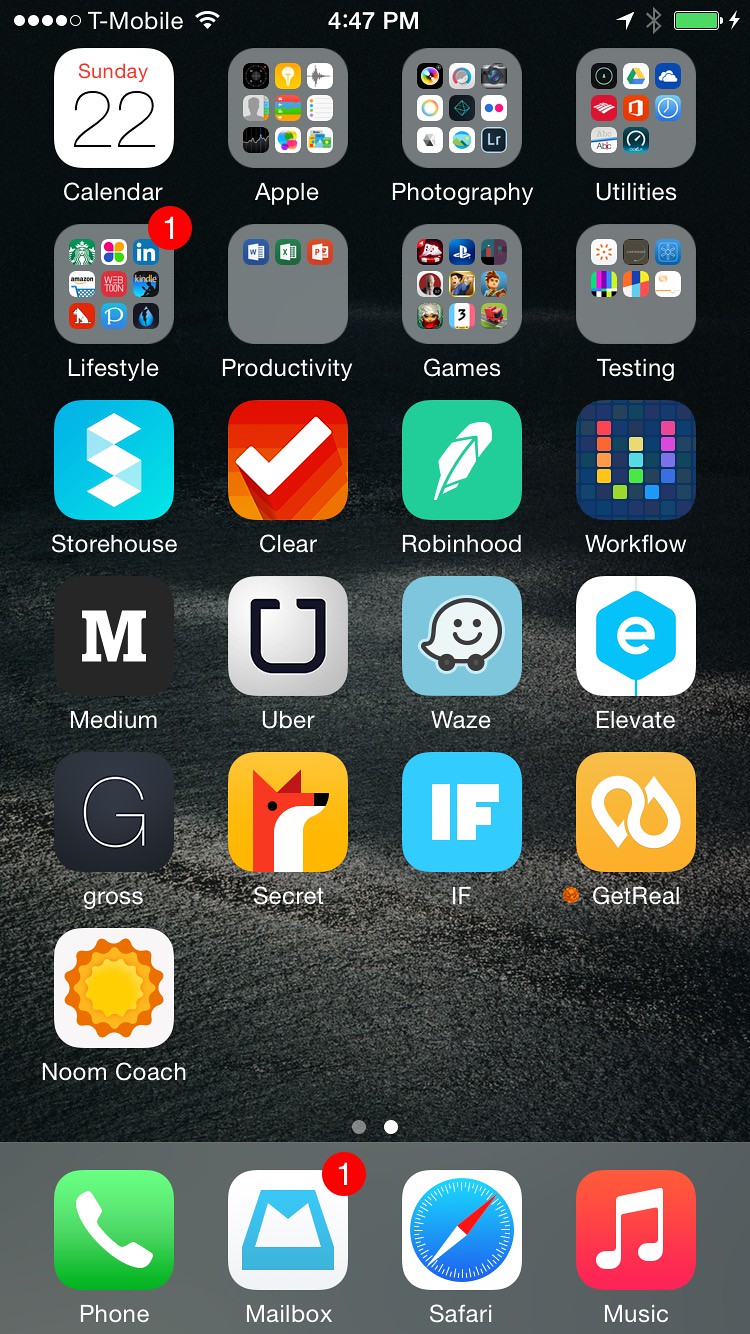A smartphone home screen is displayed, showing various app icons meticulously organized across different categories. In the top left corner, there is a "Calendar" icon. Next to it is a folder titled "Apple," containing various Apple-related icons. Adjacent categories include "Photography," "Utilities," "Lifestyle," "Productivity," and "Games." Additionally, there are folders labeled "Testing" and individual apps such as "Storehouse," "Clear," "Robinhood," "Workflow," "Medium," "Uber," "Waze," "Elevate," "Grove," "Secret," "IFTTT," "Get Real," and "Noom Coach."

At the bottom left of the screen, a green "Phone" icon can be seen, alongside a "Mail" icon showing one unread email. The "Safari" browser icon is situated next to them. Completing the row at the bottom right is the "Music" app.

The phone's lock screen still shows at the top: the carrier "T-Mobile" is displayed on the top left with three bars of signal strength. The battery icon at the top right indicates a full charge, next to which is the Bluetooth symbol. The time reads 4:47 PM.